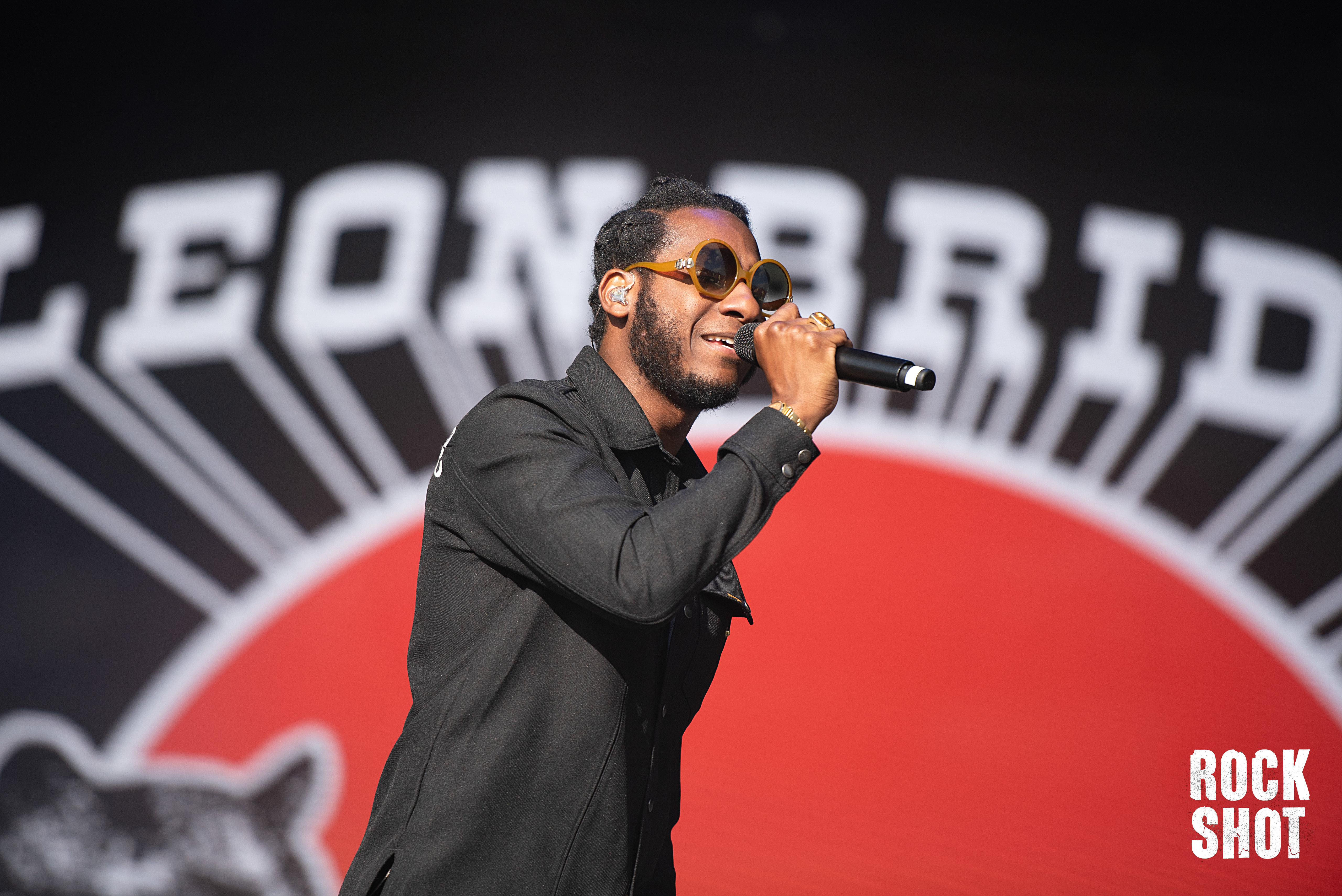The image features an African-American man with dark brown hair, braided at the top and sides, and parted. He is wearing round orange sunglasses and is captured singing into a microphone, possibly performing on a stage. He is dressed in a black button-down shirt with a black collar, featuring two buttons on the wrist of his sleeve. The man also has an earpiece in his ear, a short beard, and a clean-shaven mustache area above his lip. The stage backdrop behind him reads "Leon B-R-I-D," likely referring to Leon Bridges, with a red sun below his name on a black background. The letters of his name have stripes extending outward towards the sun, creating an impression of movement. There's also a small image of a cat in the lower left corner and the words "Rock Shop" in white text in the lower right corner. The man appears to be moving towards the right, and there is some indistinct white writing on the back of his shirt.